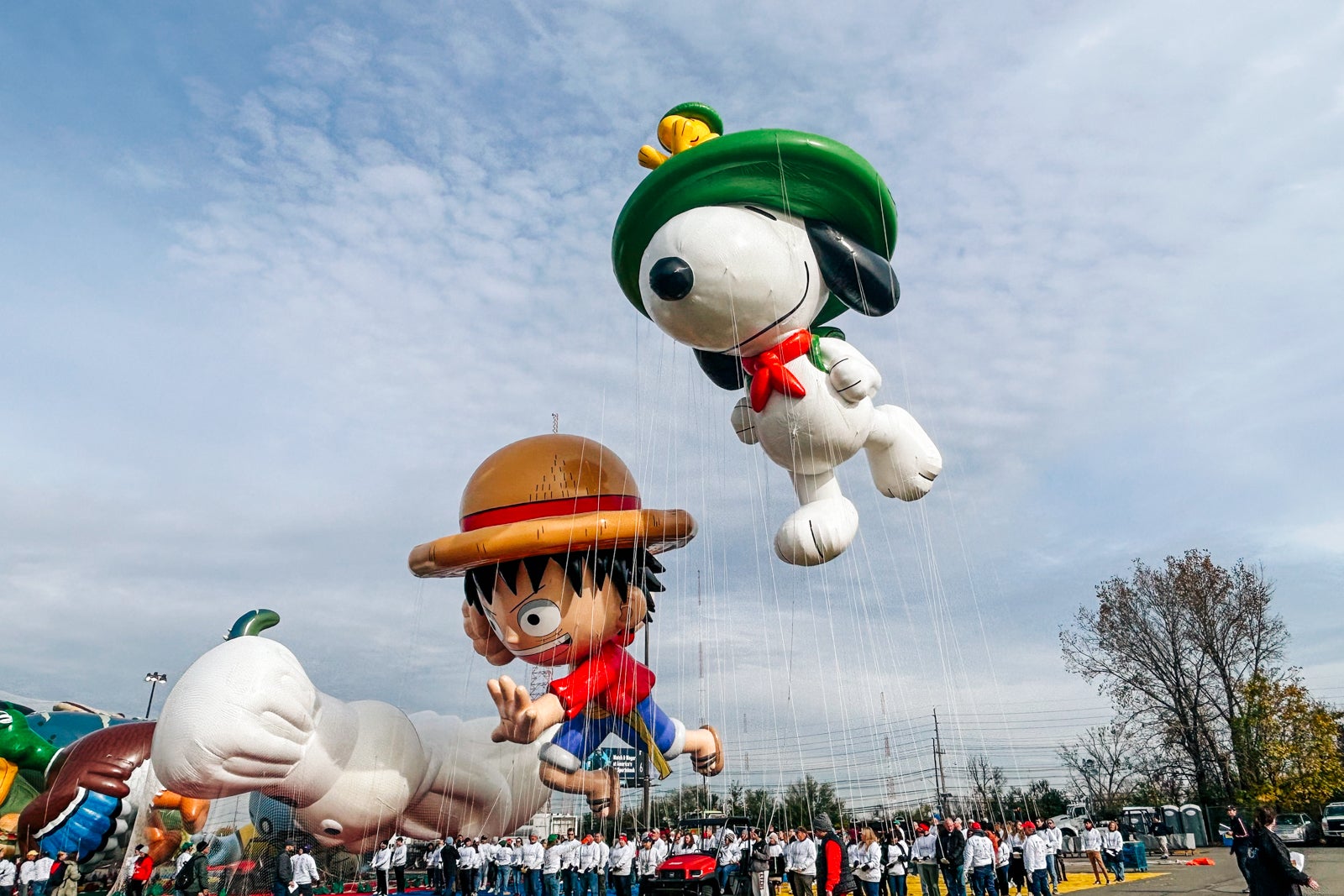On a moderately sunny, partly cloudy day, a group of people is gathered in a parking lot, preparing for a parade featuring large, well-known inflatable balloons. Dominating the scene is a high-flying Snoopy balloon, dressed in a green beret with Woodstock perched on top. Surrounding Snoopy are several other famous character balloons in various stages of inflation: the Pillsbury Doughboy, a large duck, and a cartoon figure resembling Luffy from One Piece, wearing a red shirt, denim cut-offs, a brown hat, and sandals. Numerous handlers, dressed predominantly in white tops and blue jeans, can be seen managing the strings that anchor the balloons. There's an atmosphere of anticipation as the parade participants stand ready, awaiting the signal to begin marching. This lively scene, possibly from a regional parade similar to but not as urban as the Macy's Thanksgiving Day Parade, captures the excitement of the preparatory moments just before the spectacle unfolds.